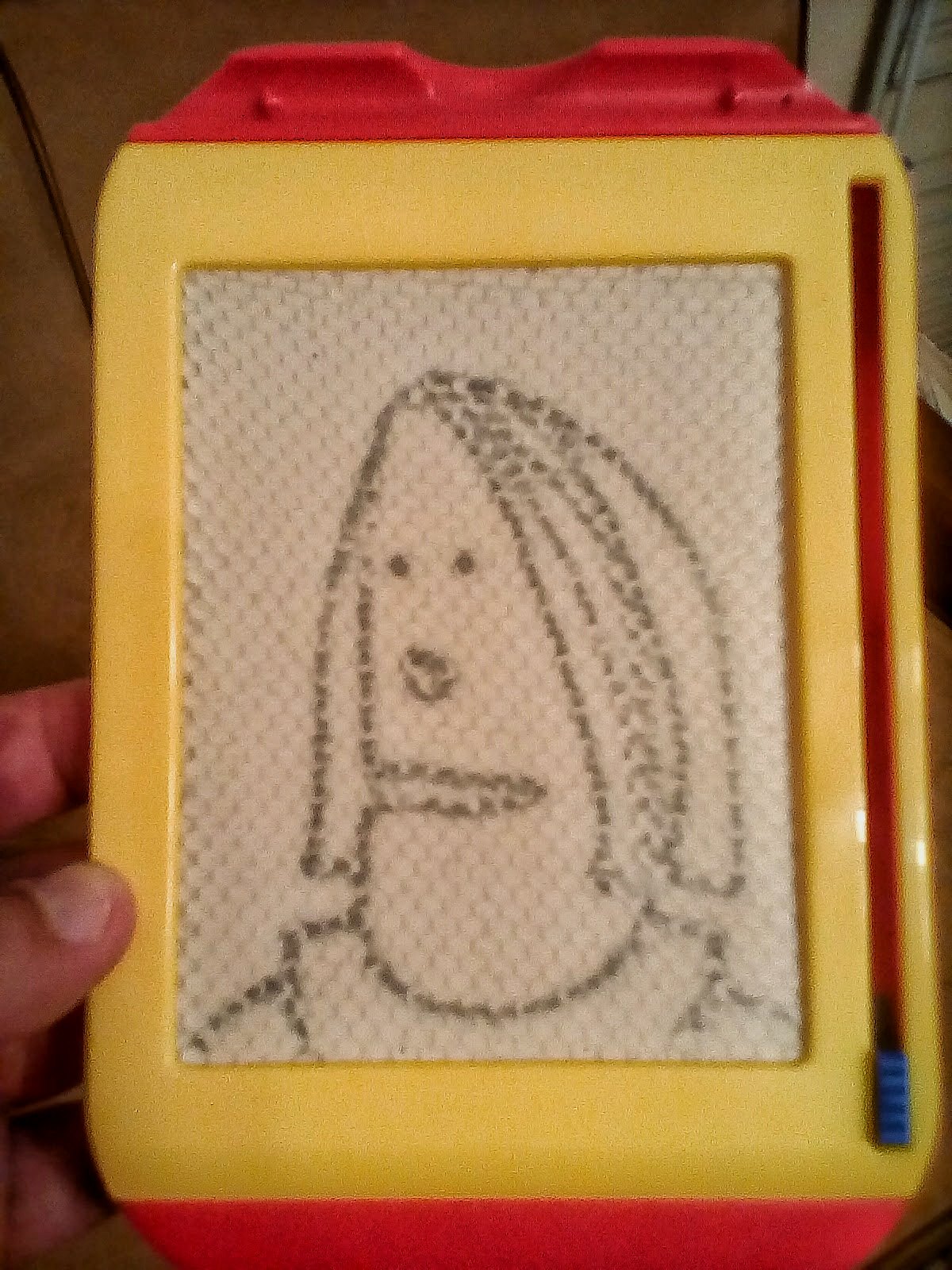The image captures a detailed indoor scene of a hand holding a small child's Etch-A-Sketch toy. The background features a dark tan or very light brown carpet in the upper left and a light tan hardwood floor in the upper right. A black extension cord runs from the left to just behind the Etch-A-Sketch. In the photo, a Caucasian hand is grasping the toy, with the thumb positioned over the white portion and the other fingers behind it.

The Etch-A-Sketch itself has a distinctive design: a red top and bottom frame, a yellow bezel with a gray inner screen, and a blue ridged piece on the right side that is used to clear the screen. The gray inset displays a very childlike, crudely drawn figure in black, facing left with a gaping mouth, a testament to the difficulty of creating art on this toy. The toy is unmistakably characterized by thin black hexagons on the screen, typical of its design. The photograph is taken in portrait mode, emphasizing the toy's rectangular shape and vibrant colors.